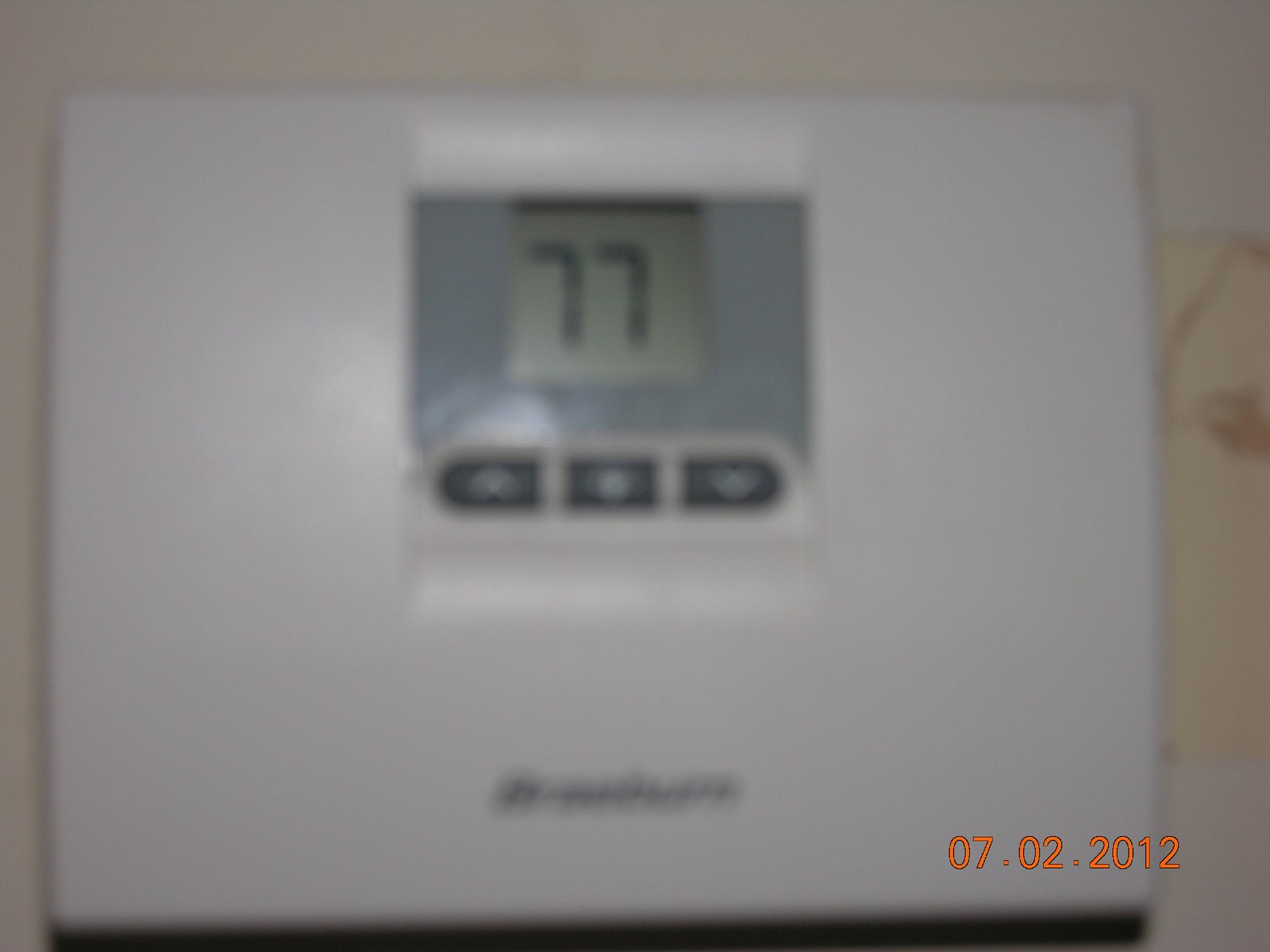In this horizontally-oriented, rectangular image, we observe a very blurred and grainy, low-resolution photograph. The lower right corner displays a digital date, "07-02-2012," in light orange text. The main subject of the image appears to be a floor scale likely used for weighing people. The scale features illegible black print on its lower center.

At the center of the scale is a digital display showing the number "77." Below this display are three rectangular black buttons, each marked with a white circle or similar symbol in their centers. Despite the scale being white, the overall look is shadowy and grainy due to the image's poor quality. The scale is placed on what seems to be a light tan tile floor, with faint horizontal lines suggesting a tiled pattern.